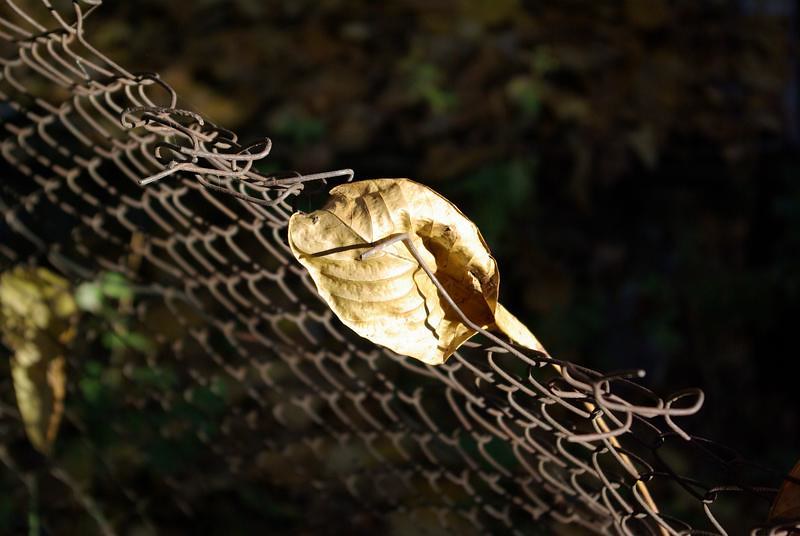In this nighttime photograph, a desiccated brown leaf clings precariously to a diagonally oriented chain-link fence. The leaf, appearing fragile and brittle, creates a striking focal point as it is illuminated by a direct light source, casting it against the surrounding shadows. The fence seems somewhat disarrayed, with chain links twisted and cut, suggesting it's either torn down or leaning. On the left side of the image, two other leaves—a green one and another transitioning to yellow-brown—are visible. Behind the fence, areas of green foliage are perceptible amidst the prevalent darkness, hinting at surrounding trees but remaining blurred and obscured by shadows. The overall dim ambiance sets a mysterious tone, accentuating the solitary spotlight on the central brown leaf.